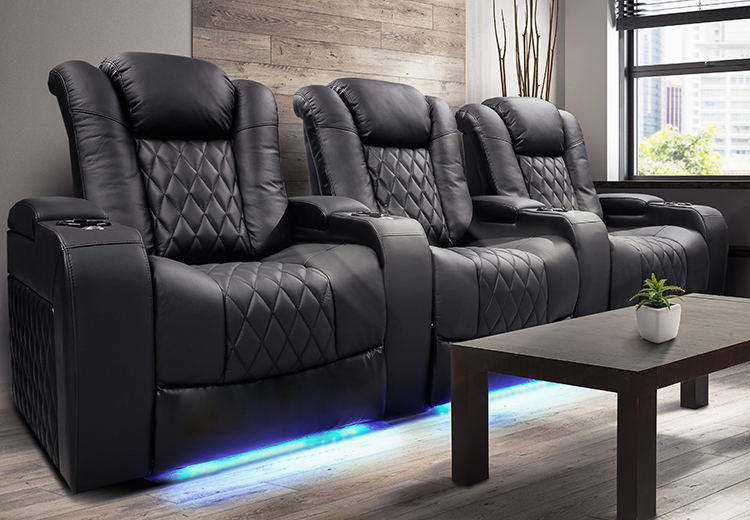The photograph captures a corner of a sophisticated living room dominated by three luxurious black leather recliners, arranged side by side in a configuration reminiscent of movie theater seating. The plush, overstuffed recliners, each featuring a pattern of indented diamonds and cup holders on their right armrests, are illuminated from beneath by a soft glow of blue neon lights. These seats rest on a sleek gray wooden floor.

In front of the seating arrangement, a dark brown walnut coffee table stands prominently, supporting a minimalist white planter with a verdant green plant. The backdrop consists of a striking contrast: vertical wooden slats occupy the middle section of the wall, flanked by off-white drywall on either side. A window to the left of the setup offers a glimpse into the urban landscape outside, with its blinds pulled halfway up, letting in daylight and revealing the top of a tree.

Additionally, a standing plant in the corner behind the leftmost recliner adds a touch of nature to the modern space, completing the serene yet sophisticated ambiance of this city living room.